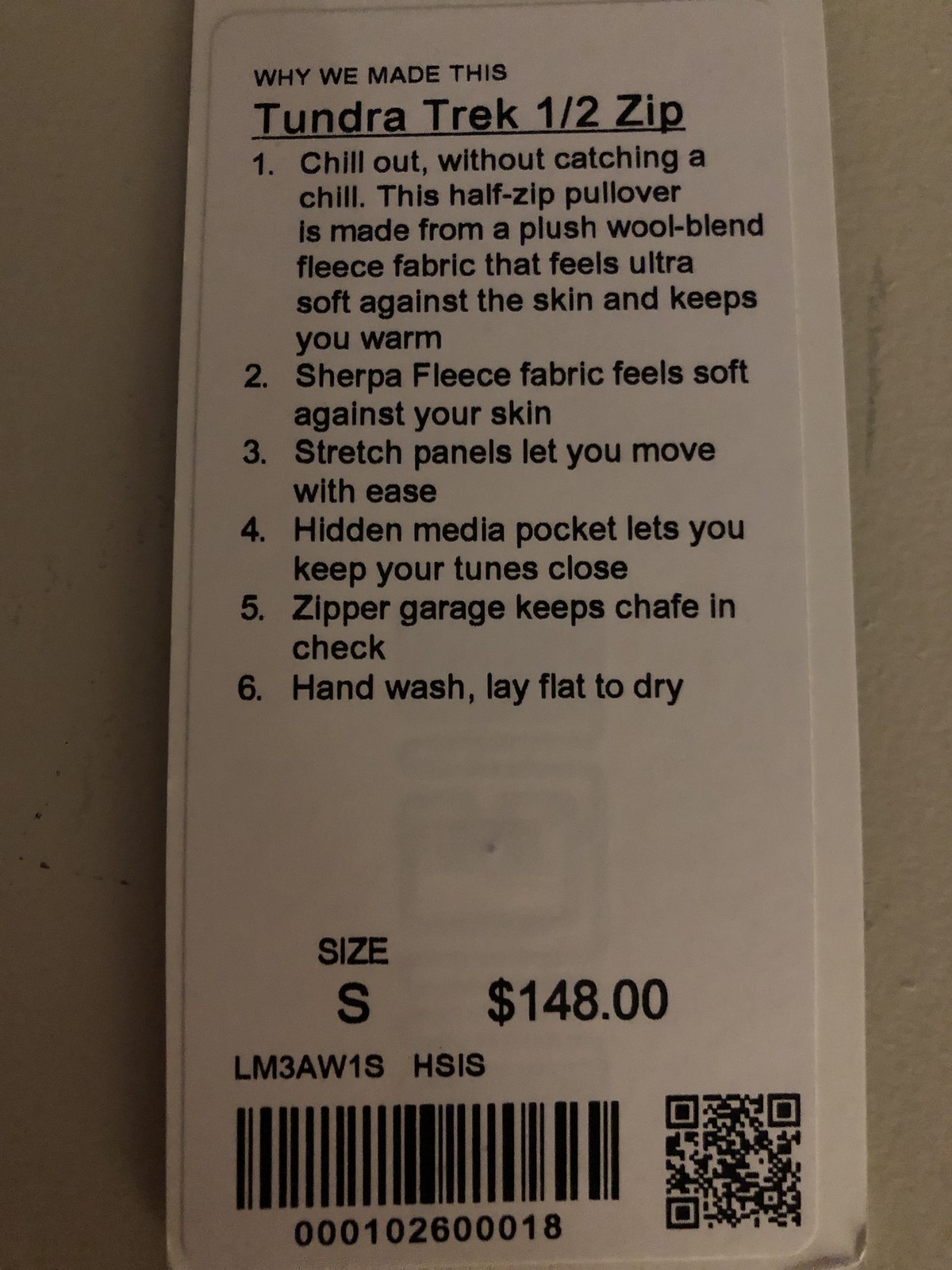This image features a white clothing tag with black text, prominently positioned in the center against a brownish off-white background. At the top of the tag, in small letters, it says, “Why we made this,” followed by larger text that reads, “Tundra Trek Half Zip.” The tag details six numbered key features of the half-zip pullover: 

1. "Chill out, without catching a chill" – this pullover is crafted from a plush wool blend fleece fabric that feels ultra-soft against the skin and keeps you warm.
2. Sherpa fleece fabric provides exceptional softness against the skin.
3. Stretch panels allow for easy movement.
4. Hidden media pockets keep your tunes close.
5. A zipper garage helps prevent chafing.
6. Care instructions specify to hand wash and lay flat to dry.

At the bottom of the tag, it indicates a size small and a price of $148. Additionally, there is a barcode with numbers underneath on the left, and a QR code symbol to the right.